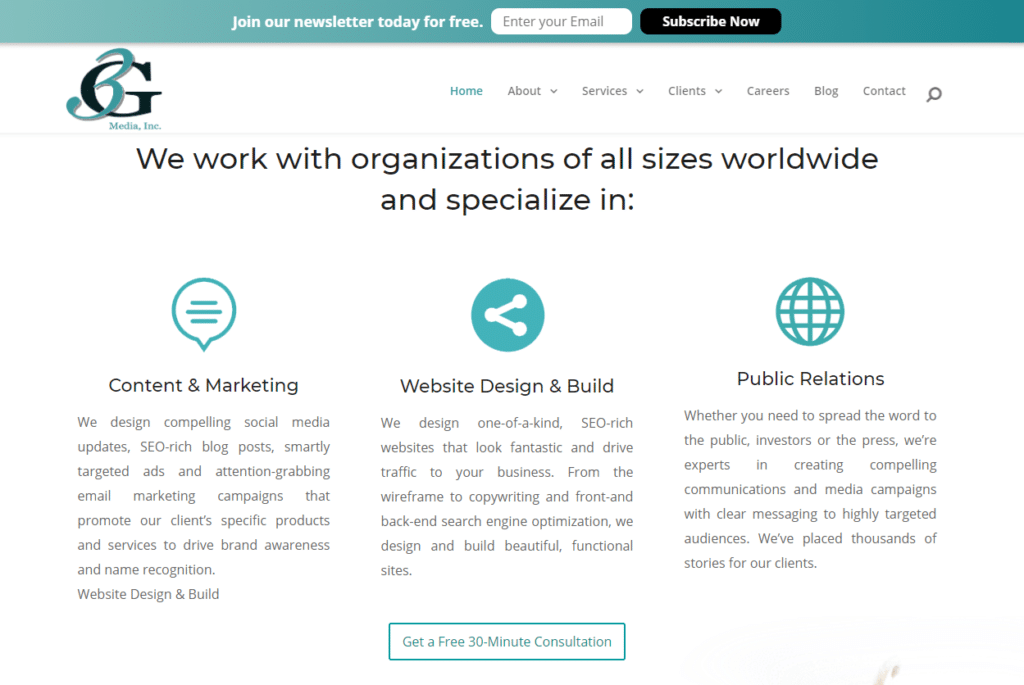Screenshot of the 3G Media Inc. Website

The screenshot depicts the homepage of 3G Media Inc.'s website. At first glance, the site features a predominantly white background accentuated by teal and black elements. The teal color is prominently used in banners, logos, and buttons, while the text is displayed in black. Notably, the design is minimalistic, lacking any photos, allowing for a clean and focused layout. 

The homepage is structured into three main columns, each detailing different specialties of the organization, such as content marketing, website design and build, and public relations. Each section is accompanied by a brief explanation of the services offered. 

A teal banner at the top inviting visitors to "Join our newsletter today for free" stands out, providing a field to enter an email address and a subscribe button. 

Navigation options are placed at the top of the page, including Home, About, Services, Clients, Careers, Blog, Contact, and a search bar. The site emphasizes its global reach and versatility, stating, "We work with organizations of all sizes worldwide."

Lastly, a prominent call-to-action button encourages visitors to "Get a free 30-minute consultation," making it easy for potential clients to engage with the company.